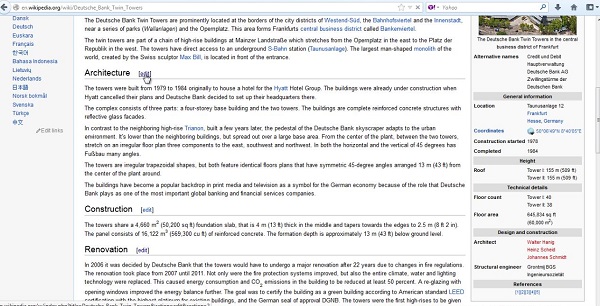This image is a screenshot from a Wikipedia article featuring the Deutsche Bank Twin Towers. The article highlights architectural details, with specific emphasis on the buildings' construction and renovation. The screenshot shows a user's mouse cursor clicking the edit button, indicating an attempt to modify or review the content. Despite zooming in, much of the text remains too small to read clearly.

Key points from the article include information about a major reconstruction initiated in 2006 due to updated fire regulations after 22 years of use. The renovation, which spanned from 2007 to 2011, involved significant upgrades to the fire protection systems as well as enhancements to the building's climate, water, and lighting technologies. These efforts successfully reduced the towers' energy consumption and CO2 emissions by at least 50%. Additionally, the re-glazing with opening windows further improved the buildings' energy efficiency. The overarching goal of the renovation was to achieve certification as a green building according to the American LEED standards.